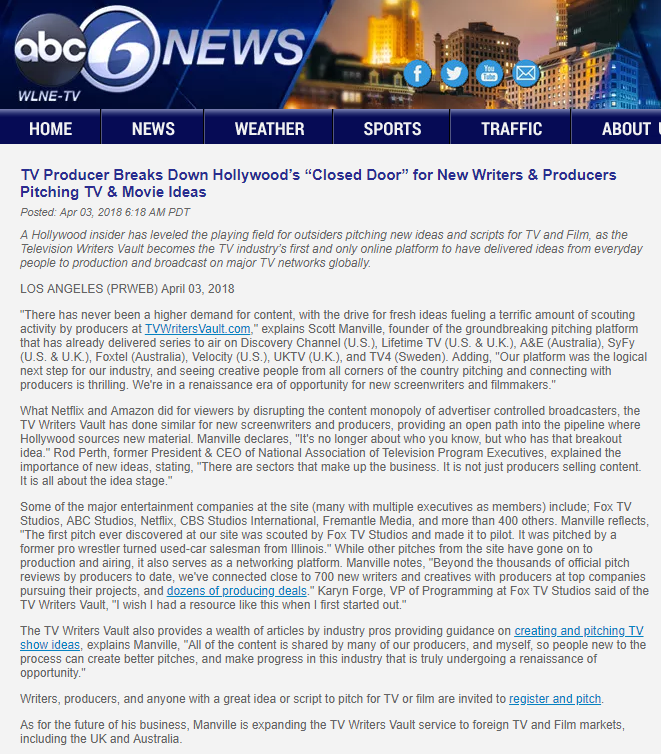**Screenshot of a News Article on ABC6 News WLNE-TV**

**Title:** "TV Producer Breaks Down Hollywood's Closed Door for New Writers and Producers Pitching TV and Movie Ideas"

A detailed screenshot captures a news article from ABC6 News WLNE-TV. The headline reports on a significant development for aspiring writers and producers in the entertainment industry. It reads: "TV Producer Breaks Down Hollywood's Closed Door for New Writers and Producers Pitching TV and Movie Ideas." The article highlights how a Hollywood insider has democratized the pitching process, enabling outsiders to present their ideas and scripts to TV and film producers. This new opportunity is made possible by a groundbreaking platform, TVwritersvault.com, which has become the industry's first and only online service to successfully deliver everyday people's ideas to major TV networks globally.

The article further details, below a subheading, "Los Angeles PRWEB, April 3rd, 2018," that the demand for fresh, innovative content is at an all-time high. Scott Manville, the founder of TVwritersvault.com, explains that the drive for unique ideas has fueled significant scouting activity by producers on the platform. Manville's brainchild has already helped launch series on prominent networks including the Discovery Channel (U.S.), Lifetime TV (U.S. and U.K.), A&E (Australia), Syfy (U.S. and U.K.), Foxtel (Australia), and Velocity (U.S.).

This detailed caption showcases the transformative impact of TVwritersvault.com in making Hollywood more accessible to fresh talent from around the world.